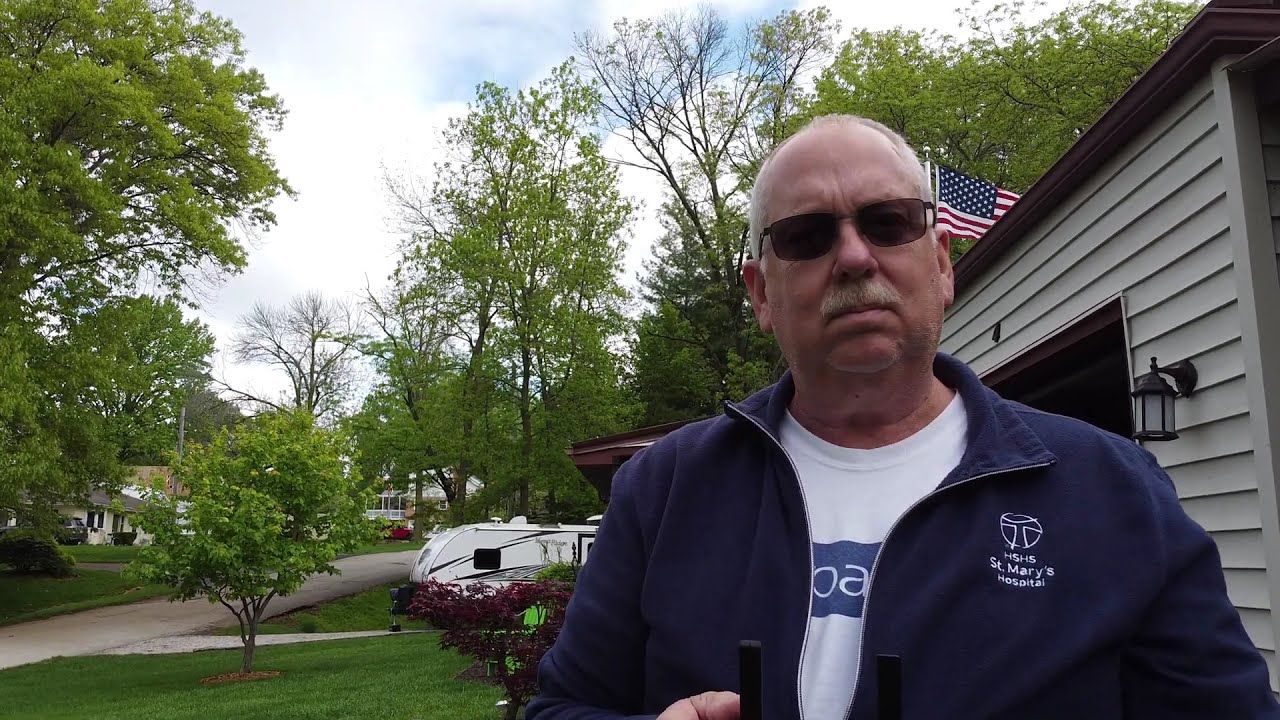The photograph captures an older man with short white hair and a light-colored mustache, wearing dark sunglasses. He is dressed in a white shirt with a partially unzipped navy blue jacket bearing the emblem and name "HSHS St. Mary's Hospital" on the left chest. He stands close to the camera, roughly from the waist up, set against the backdrop of a house with a white exterior and a brown roof. To the right of the man, beige vinyl siding of a garage or house is visible along with an old-style lantern sconce. Peeking into the scene from the right side is a motorhome in the driveway. Behind the man's head, an American flag waves in the breeze, and the background reveals a lone tree in his yard, along with glimpses of a roadway and additional houses partially obscured by trees to the left.